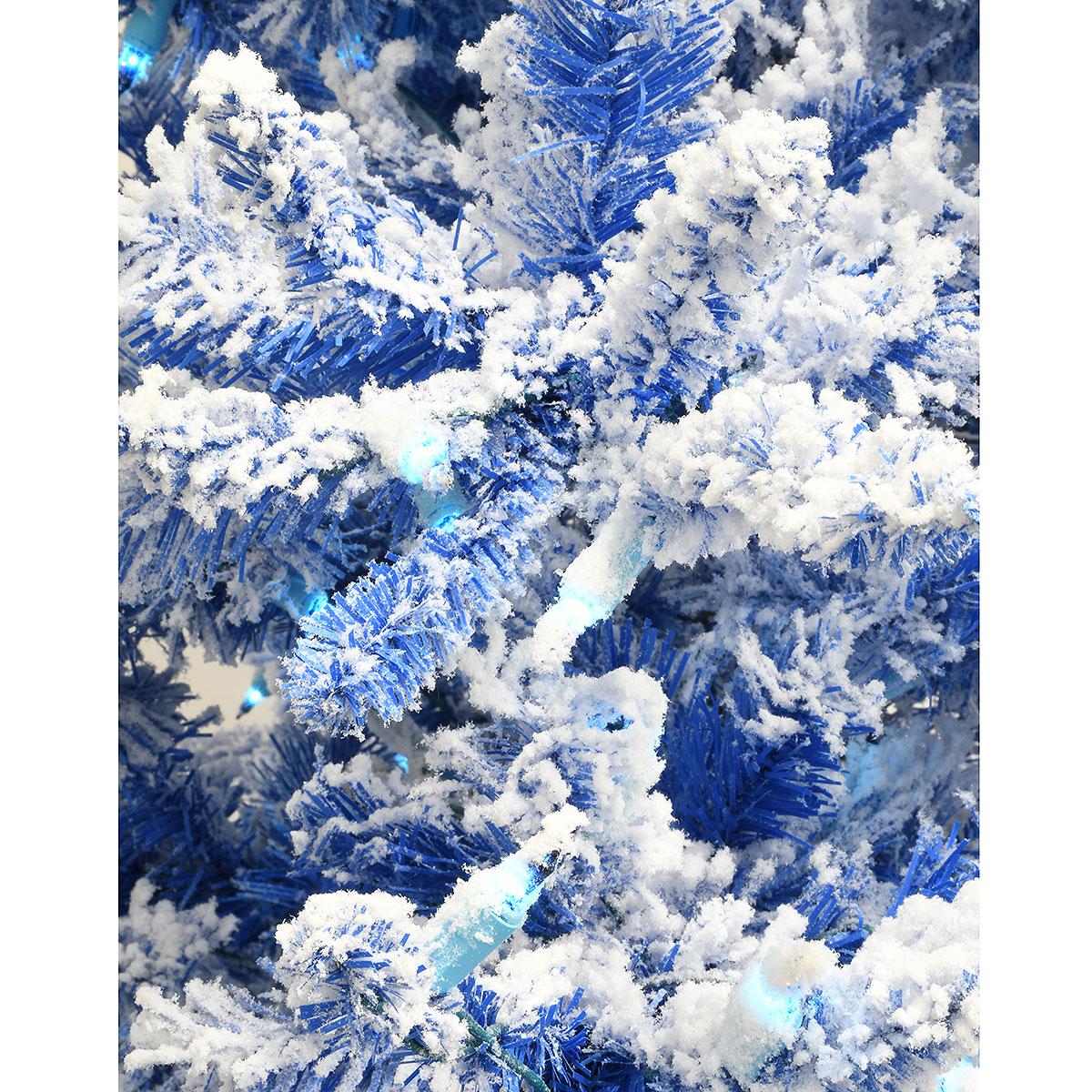This color photograph, taken in portrait orientation, showcases a centrally positioned artificial Christmas tree with short needle pine branches predominantly blue in color. The tree is adorned with light blue LED lights, spread evenly from the bottom left to the top left, enhancing its blue wintery aura. White flocking material, mimicking snow, is delicately applied to the ends of the branches, adding a frosted, snow-like effect. There are tightly packed branches, with the background mostly obscured but revealing a gray wall. Below the tree, towards the center left, a light blue plastic device, illuminated and possibly a plug, is visible. Additionally, a twisted metal piece can be seen next to one of the lights in the image, further contributing to the tree's intricate and festive details.